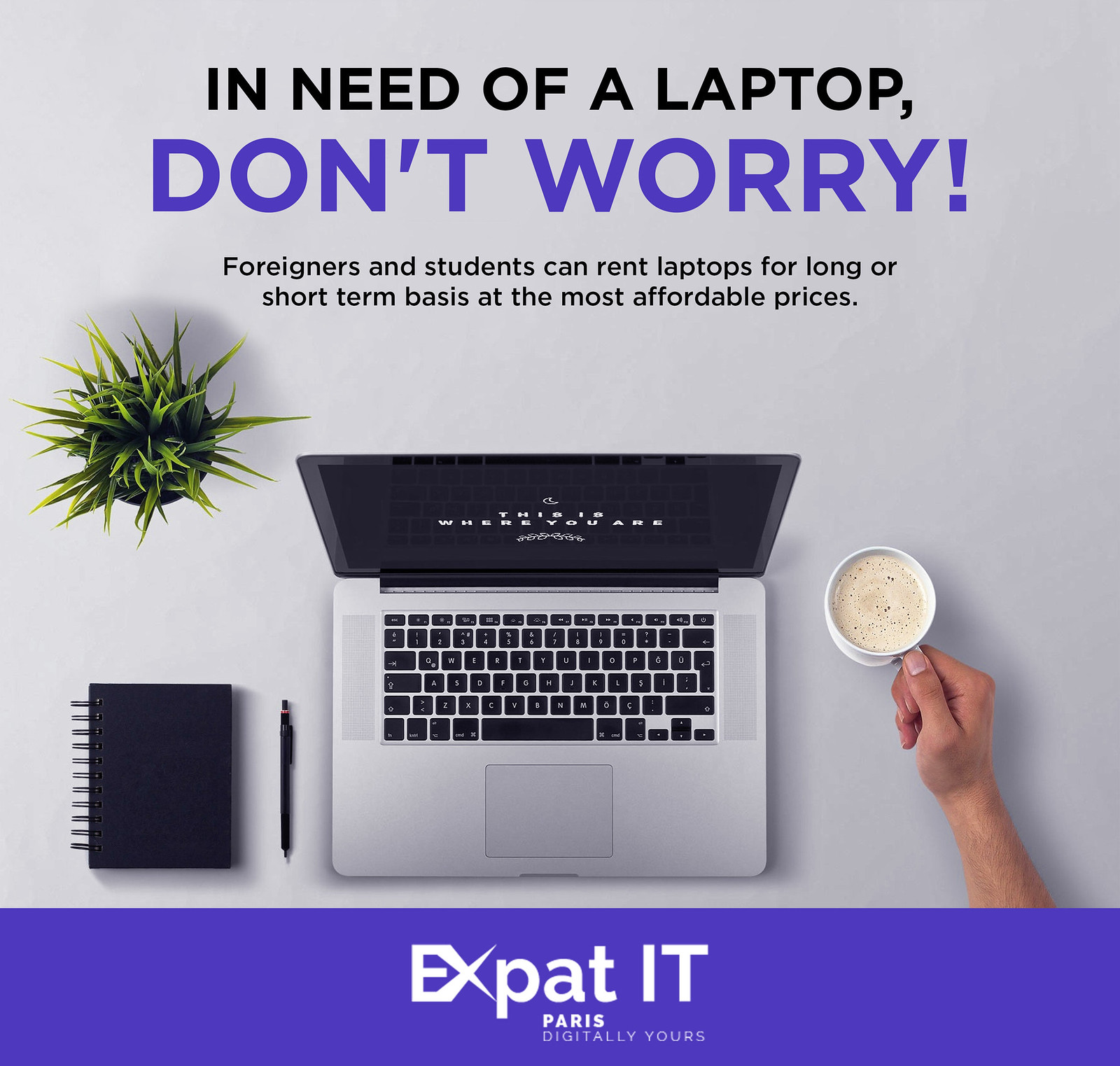The square poster features a grey background, depicting a scene on a grey table. At the top, it reads in bold black text, "In need of a laptop," followed by larger blue text, "Don't worry!" Beneath this, in smaller black print, it states, "Foreigners and students can rent laptops for a long or short term basis at the most affordable prices."

The central image showcases an open silver laptop with a black keyboard, its screen displaying white text, viewed from an angle slightly above. To the left of the laptop is a green, spiky plant, a black pen, and a black notebook. On the right side of the laptop, an arm extends from off-screen, holding a white mug filled with a foamy beverage.

At the bottom of the poster, a wide blue band features the text "Expat IT Paris" in white, followed by "digitally yours." This advertisement is designed to offer reassurance and practical information for potential laptop renters.